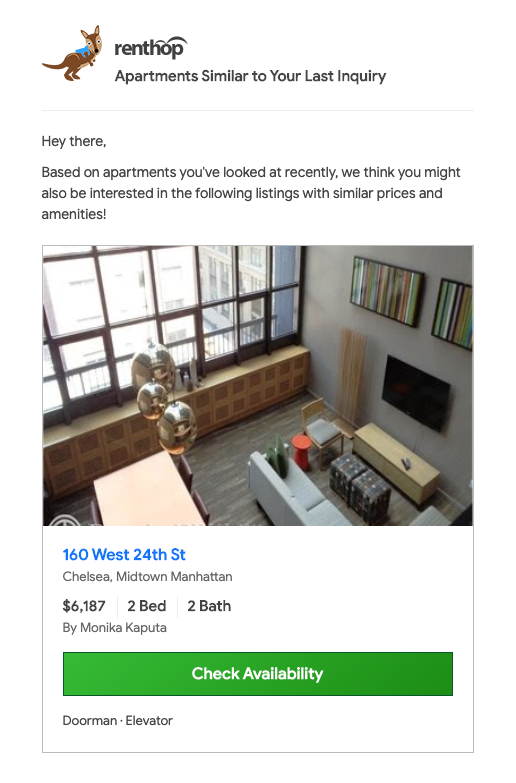This image is a screenshot from the RentHop application. The background is predominantly white with black text, except for a prominent section featuring blue text. In the top left corner, there's a cartoon drawing of a kangaroo wearing a blue sack on its back, signifying the RentHop brand. Next to the kangaroo, the text reads: "RentHop - Apartments similar to your last inquiry."

Below this header, another text passage says, "Hey there, based on apartments you looked at recently, we think you might also be interested in the following listings with similar prices and amenities." 

The main part of the image showcases a photograph of a room in an apartment, characterized by large windows, pictures, and TVs mounted on the wall, and hardwood floors. Under this image, the blue-colored text highlights the property details: "160 West 24th Street, Chelsea, Midtown, Manhattan, $6,187. Two bedroom, two bathroom by Monica Caputa." Additionally, a "Check Availability" button is visible beneath the property description, along with icons indicating the presence of a doorman and an elevator.